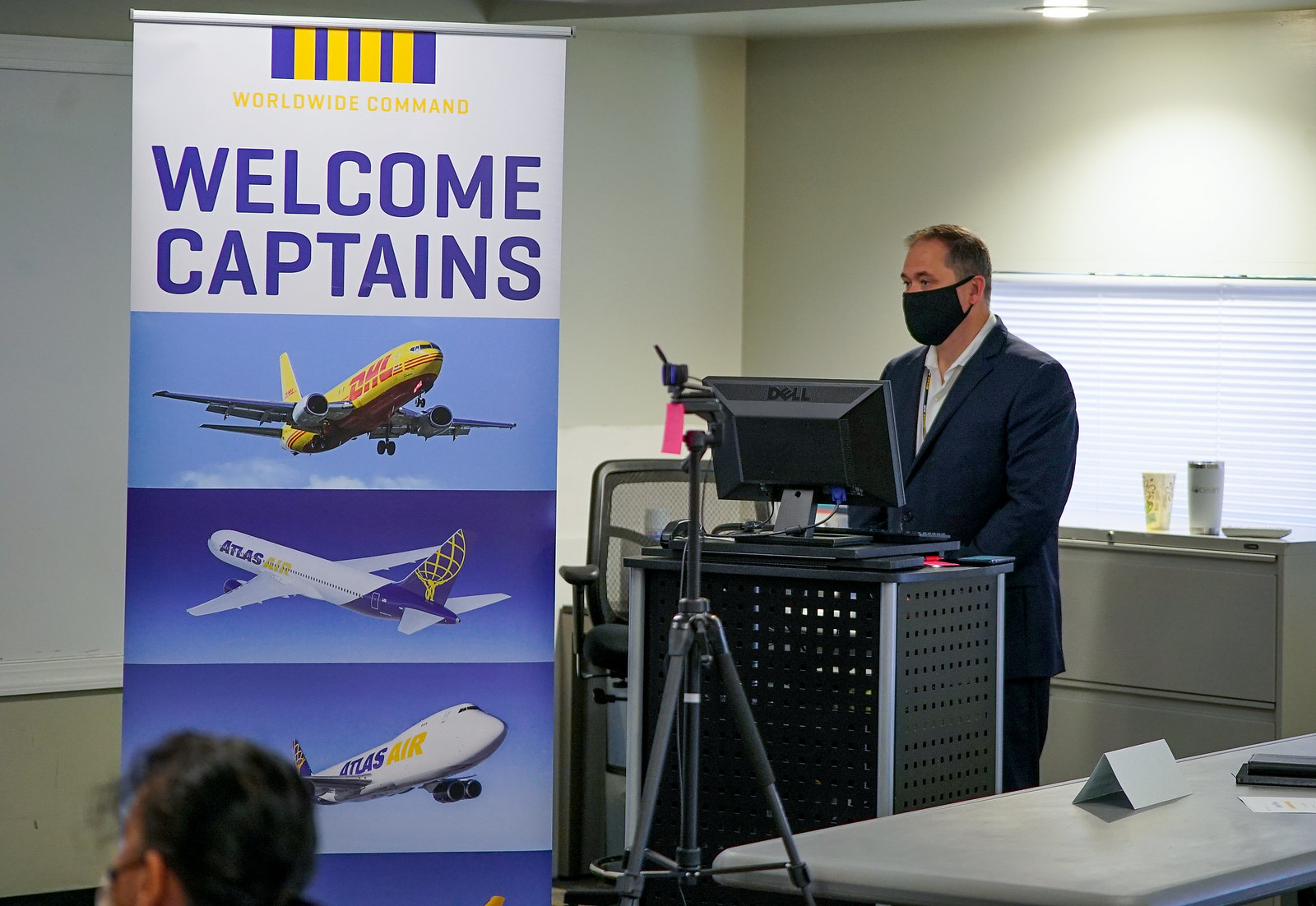The image depicts a man, who appears to be in his 40s, wearing a suit jacket, white shirt, and a black mask, standing at a podium, delivering a presentation. He has short, dark hair and is positioned behind a podium that has a computer with a phone mount draped over its edge. The backdrop features a white wall with a prominently placed banner on the left reading, "World Wide Command" in yellow at the top, followed by "Welcome Captains" in bold, capitalized blueprint text. The banner is accented with yellow and blue stripes and displays three images of airplanes in flight, representing Atlas Air and DHL. This setting suggests a conference or a training session for airplane captains. Another masked attendee, possibly looking at a presentation on a screen or a PowerPoint, is partially visible, indicating the ongoing nature of the event.